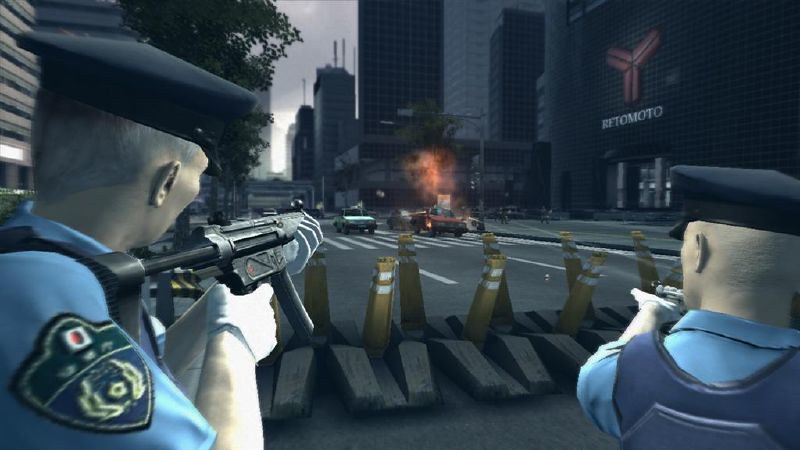A tense standoff unfolds in this video game screenshot set within a bustling cityscape. Flanking both the left and right corners of the image are two determined law enforcement officers, each brandishing firearms aimed at a distant vehicle. They are positioned behind a formidable riot barrier adorned with bright orange and white-striped poles, interspersed with bricks and other makeshift obstacles to deter intruders. The setting is framed by towering buildings that line both sides of the street, creating a claustrophobic urban canyon. Ahead, in the crosswalk, several vehicles are caught in the line of fire. The overcast sky looms ominously overhead, devoid of any trace of blue, adding to the gritty, high-stakes atmosphere of the scene.